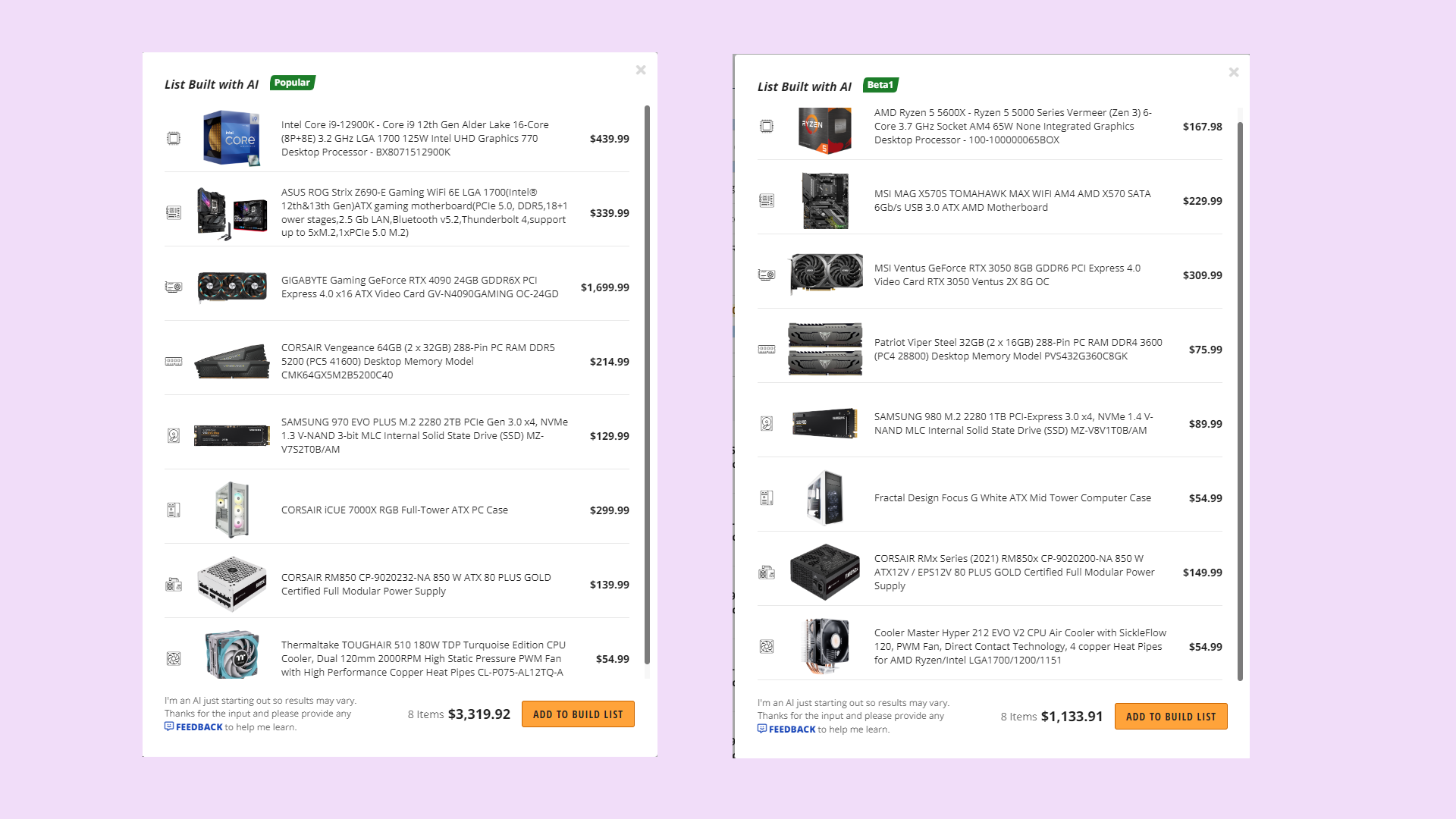This image shows two pages displayed side-by-side, set against a pink background that separates the two pages slightly. The pages themselves are white, each featuring an item that appears to be a computer component. Both pages have a title in the upper left corner that reads "List built with AI".

On the left page, just to the left of the title, there's a green box labeled "Popular." The main product listed on this page is an Intel Core desktop processor, priced at $439.99.

On the right page, the title "List built with AI" is mirrored to the right, with a label to the left that reads "Beta." The primary item on this page is an AMD Graphics processor.